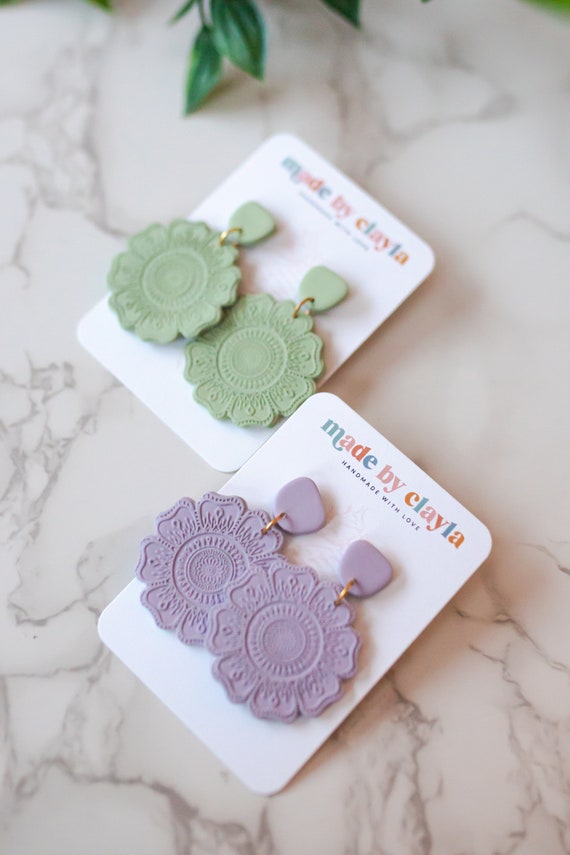This color close-up photograph features two pairs of intricately designed earrings displayed on a white, marbled surface. Each pair of earrings is mounted on a white card that reads "Made by Clayla, handmade with love" in multi-colored and black text. The top card showcases a pair of mint green earrings, while the bottom displays the same design in a light lavender hue. Both sets of earrings are crafted from a material that could be clay, given the name Clayla, with an elegant floral motif imprinted into them. The earrings consist of a small circular piece that attaches to the ear, linked with a brass or gold hoop to a larger, flower-shaped dangling portion. The background also features a few leaves from a plant peeking in at the top of the image, contributing to the composition's natural and artisanal aesthetic.